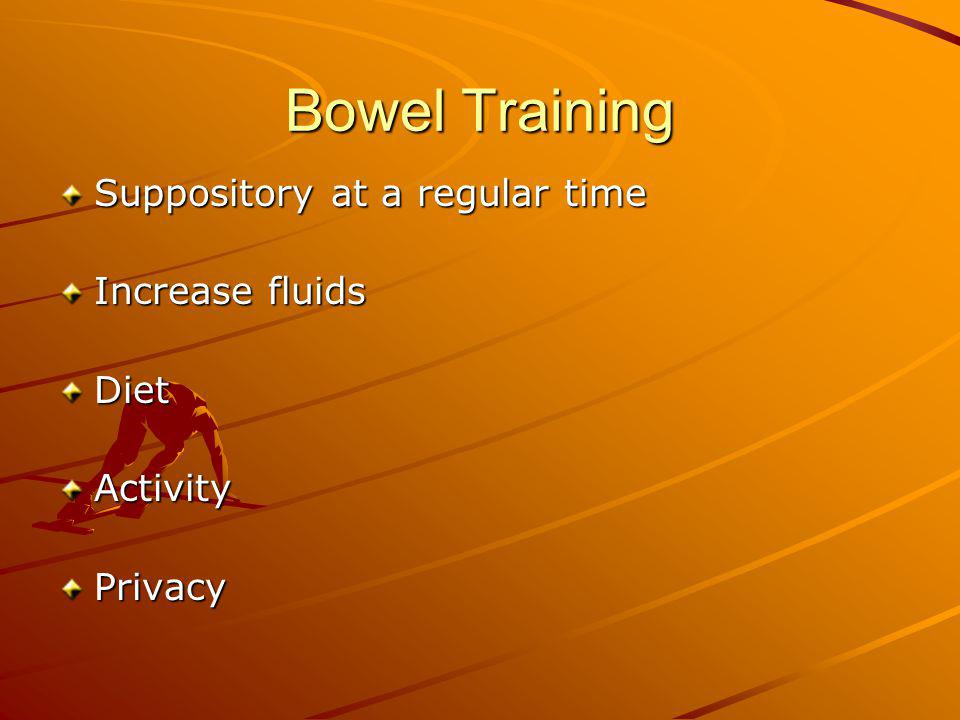The image features a slide with an orange background, depicting a person positioned at the starting blocks of a racetrack, specifically in the fourth lane, facing away from the camera. The slide is designed in a PowerPoint presentation style. At the top center, a yellow headline reads "Bowel Training." Beneath it, five bullet points in white text with yellow bullets list the following: "Suppository at a regular time," "Increased fluids," "Diet," "Activity," and "Privacy." The racetrack background has eight lanes, with lines ranging from darker brownish-gray to yellow and black, and gives a sense of an outdoor setting, though the overall image appears to be computer-generated. The runner, positioned at the bottom left corner of the image, is alone and poised to start a race.